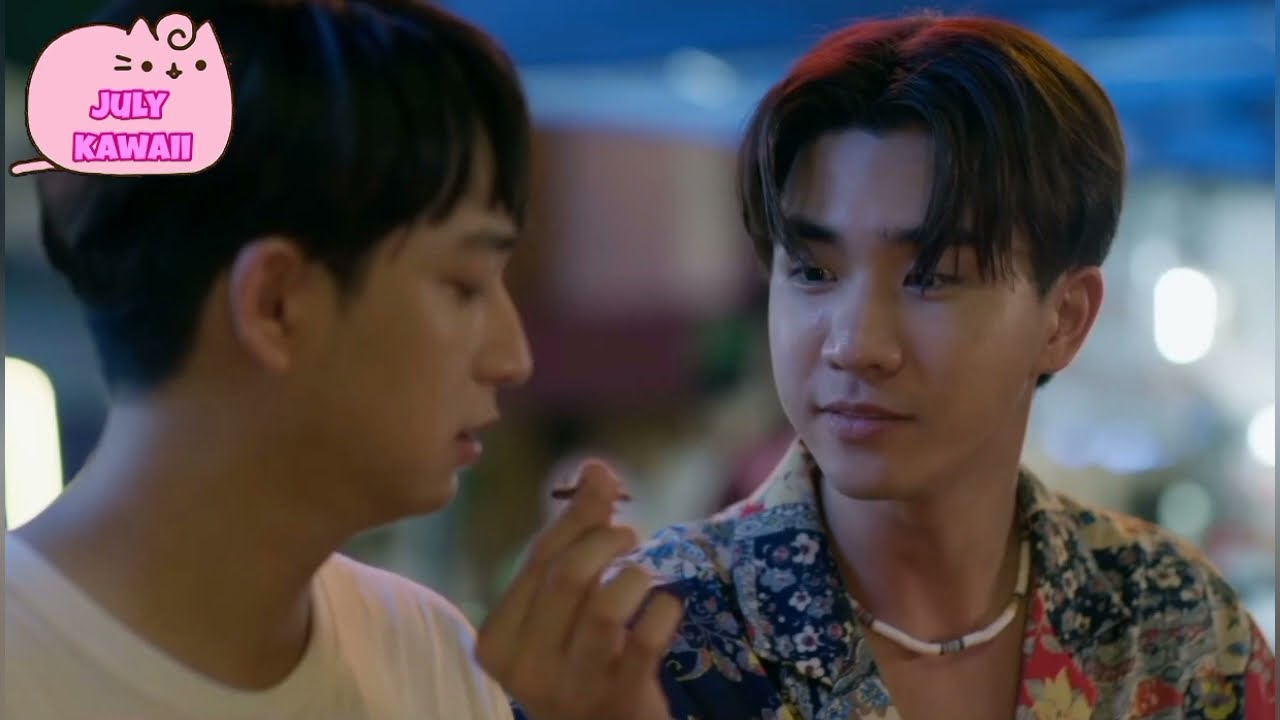In this detailed and descriptive image, we see two young Asian men, both probably teenagers, standing together. The teenager on the right is wearing an unbuttoned, floral-printed shirt, revealing a white, tight necklace around his neck. He has black hair with bangs that partially cover his eyes but are parted in the middle. He appears to be almost smiling as he holds up an object – possibly a marijuana joint or a piece of food – between his fingers, offering it to the other teen. The teenager on the left, dressed in a simple white t-shirt and with short black hair, looks apprehensive as he gazes down at the object being handed to him, yet he has not reached out to grab it. The background of the image is blurred, possibly suggesting an indoor setting like a restaurant, although the beachy attire of the teenagers hints at a tropical location. In the upper left corner, there is a simplistic, cartoon-style pink cat with whiskers, and beside it, the pink text reads "July Kauai," indicating that this scene might be taking place in Hawaii.